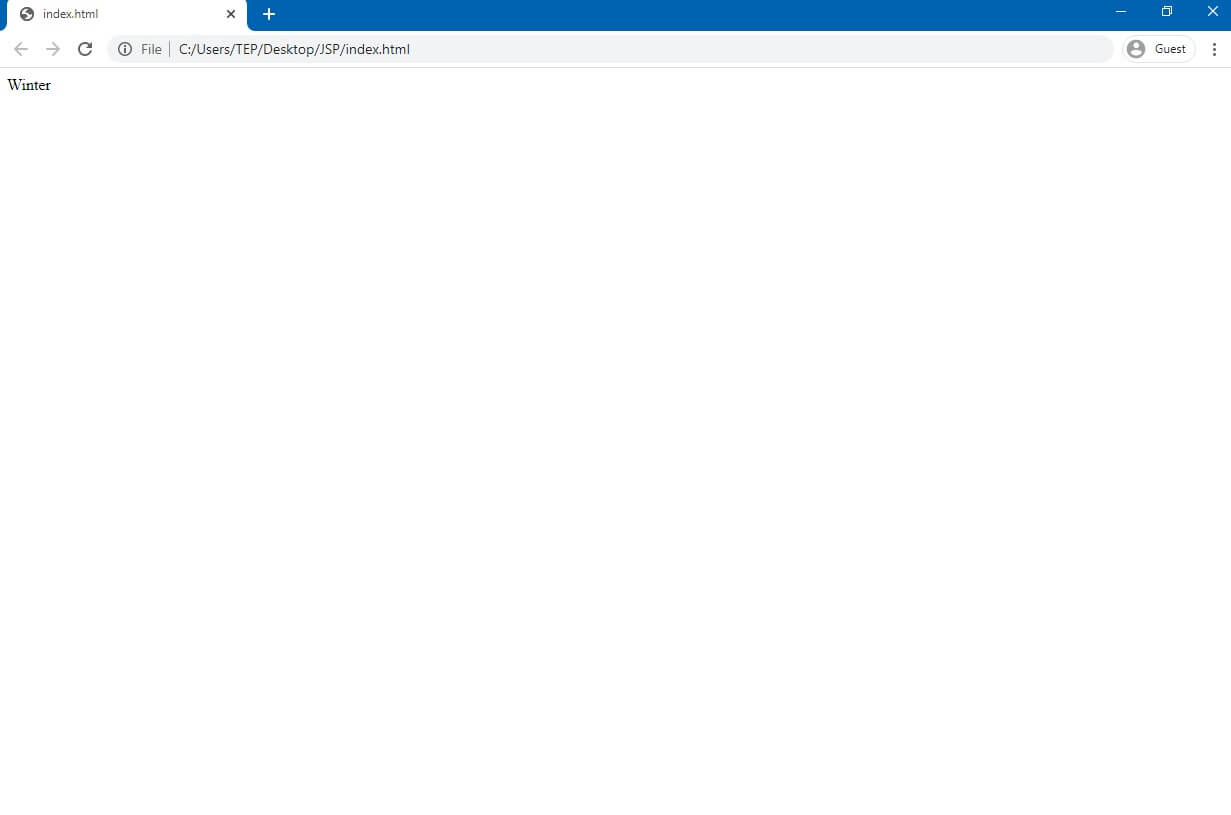This image depicts a screenshot with a predominantly white background. At the top of the screenshot, there is a blue banner. On the left side of the blue banner, a smaller white banner displays the black text "index.html." On the far right of the blue banner, there are three icons: a minus sign, a page icon, and an X.

Immediately below the blue banner lies the address bar. The address bar begins with navigation icons on the left, including left and right arrows, an undo icon, and a file icon. The address bar itself shows the following path: "C:/Users/TEP/Desktop/JSP/index.html." On the right side of the address bar, there is a circular image of a person, labeled with the word "guest" in gray text, followed by a vertical ellipsis represented by three gray dots.

Proceeding further down, a light gray horizontal line separates the address bar from the content below. On the left side of the subsequent section, black text reads "winter."